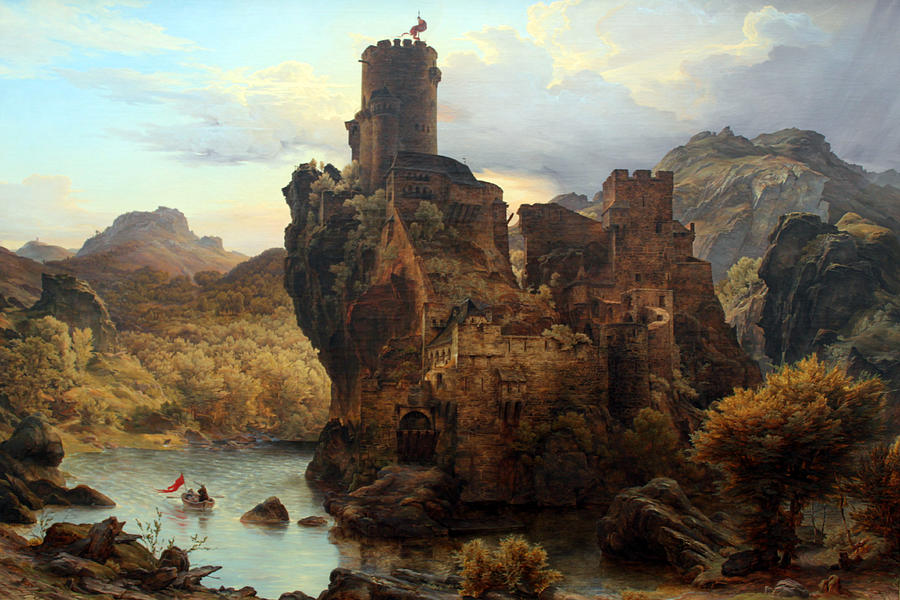The image is an old painting depicting a majestic and rugged landscape. At the center, a grand castle emerges from a cliff rock formation, rising from a murky brown and bluish lake. The castle is a complex structure made from stone or brick, featuring both rocky and castle walls. It boasts a very tall cylindrical tower topped with a red flag. The castle's architecture includes various levels and towers, both circular and rectangular, with brown doors and empty window areas. Green plants and trees cling to the side of the castle's stone walls, adding a touch of nature to the fortress.

At the base of the cliff, near the water, trees and bushes in hues of brown, green, and reddish-orange frame the scene. There is a tiny, brown rowing boat with two people on board, also flying a red flag. Surrounding the central rocky precipice are rugged mountains and dense forests that stretch into the background beneath a sky that transitions from blue with white clouds to a grayish tone on the right. This painting, likely done on canvas, beautifully captures the rough, rocky landscape and the imposing, isolated castle rising majestically above the tranquil waters.